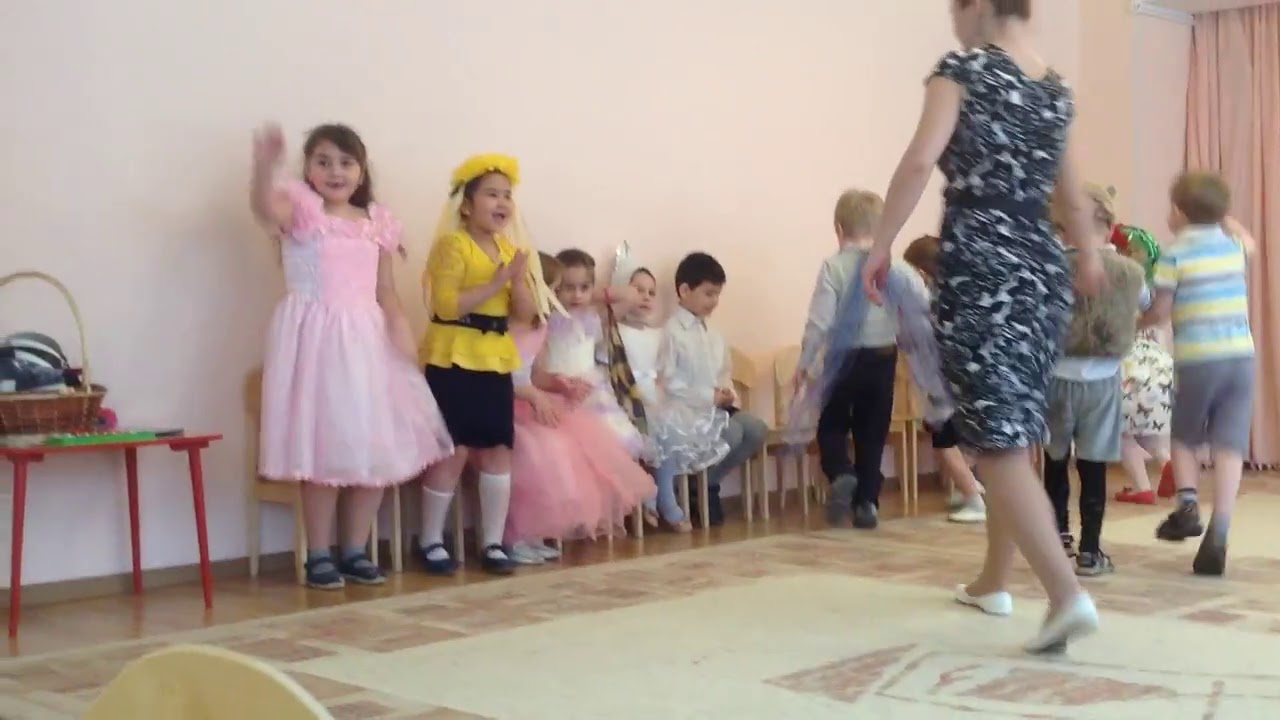In the photograph, a group of children are seated on tiny chairs along a pink wall adorned with pink curtains, with a peach and tan-colored carpet underfoot. At the center of the room, a woman in white skimmer flats and a blue, white, and black dress walks towards the children, appearing to coordinate their activities. The children are dressed up in various costumes and outfits; notably, one girl wears a pink dress, and another wears a yellow top with a black skirt, complete with a yellow-flowered wreath on her head and knee-high white socks. A boy in formal clothes with wings is also present, adding to the theatrical atmosphere that suggests a rehearsal for a play. On the far left, there is a red and green table with a basket filled with items, and on the far right, a long pink curtain hangs. The scene is vibrant and lively, capturing the organized chaos of children engaged in imaginative play.